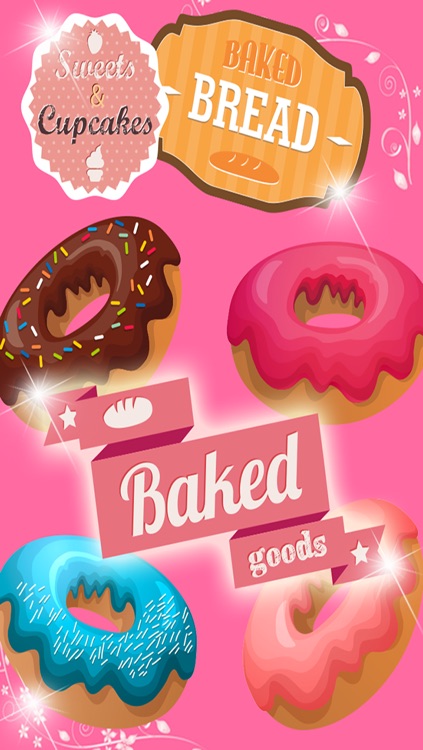The image appears to be an advertisement for baked goods, presented in a vertically oriented, column-style box with a bright pink background. At the top left, a white petal-shaped graphic with a pink overlay contains the text "Sweets and Cupcakes." Adjacent to this, on a black striped background, the words "Baked Bread" are displayed in white font. Below, there are illustrated doughnuts: one with chocolate frosting and colorful sprinkles, and another with pink frosting. In the middle of the image, a white ribbon-like banner on the pink background prominently features the text "Baked Goods." Toward the bottom, there are more doughnuts – one with blue frosting and another with light pink frosting. The doughnuts are depicted in a colorful, animated style rather than as real, photographic treats. Scattered throughout the image are drawings of loaves of bread and ice cream, enhancing the overall theme of assorted baked delights.